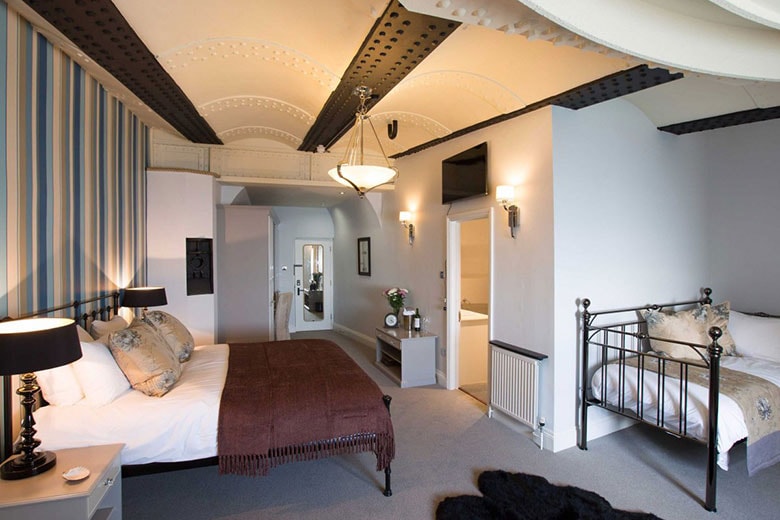The image showcases a detailed and unique hotel room within the converted 19th-century No Man's Fort in Portsmouth, which serves as a virtually private island for rent. The room features an industrial theme highlighted by an arched ceiling with black steel beams, white riveted girders, and off-white dotted patterns. The interior is illuminated by several turned-on lights, including a black lamp on a nightstand and sconces flanking a doorway leading to a bathroom.

On the right side, a day bed made up with white sheets, a tan blanket, and tan throw pillows adds comfort and style. Adjacent to it, there's a queen or king-size bed adorned with white sheets, tan and white pillows, and a half-folded dark brown fringed blanket. Behind the bed, vertical striped wallpaper in gray, blue, and cream hues enhances the decor.

A flat-panel TV is mounted above the bathroom doorway on the right wall, accompanied by a small radiator heater beneath it. The carpet adds coziness with its gray hue, complementing the room's serene ambience. Additionally, a small table to the left of the bathroom holds an ice bucket, bottle of wine, and a floral arrangement, contributing to the sophisticated yet welcoming atmosphere.